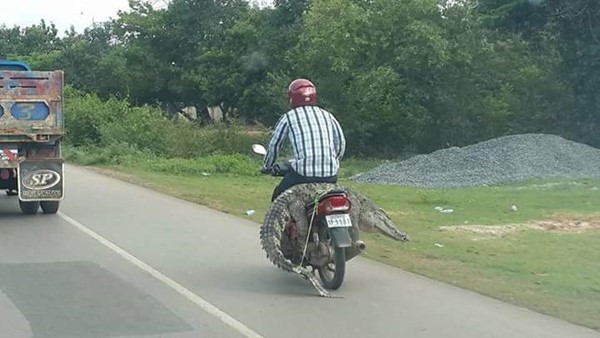In this intriguing photograph, a person is seen riding a motorcycle along the shoulder of a road with a strikingly unusual passenger—a sizable alligator draped over the back of the bike. The rider, identifiable by a red helmet and a long-sleeved shirt featuring black and blue stripes, pairs this with blue jeans. The alligator's head protrudes to the right side while its tail extends to the left, noticeably dragging along the asphalt. To the left of the rider, a truck can be seen in the adjacent lane, suggesting they are both heading in the same direction. On the right side of the road, the scenery includes a grassy area transitioning into a pile of rocks, eventually leading to a distant treeline. This unexpected and somewhat surreal scene captures a moment of curiosity and daring against a backdrop of a typical roadway environment.